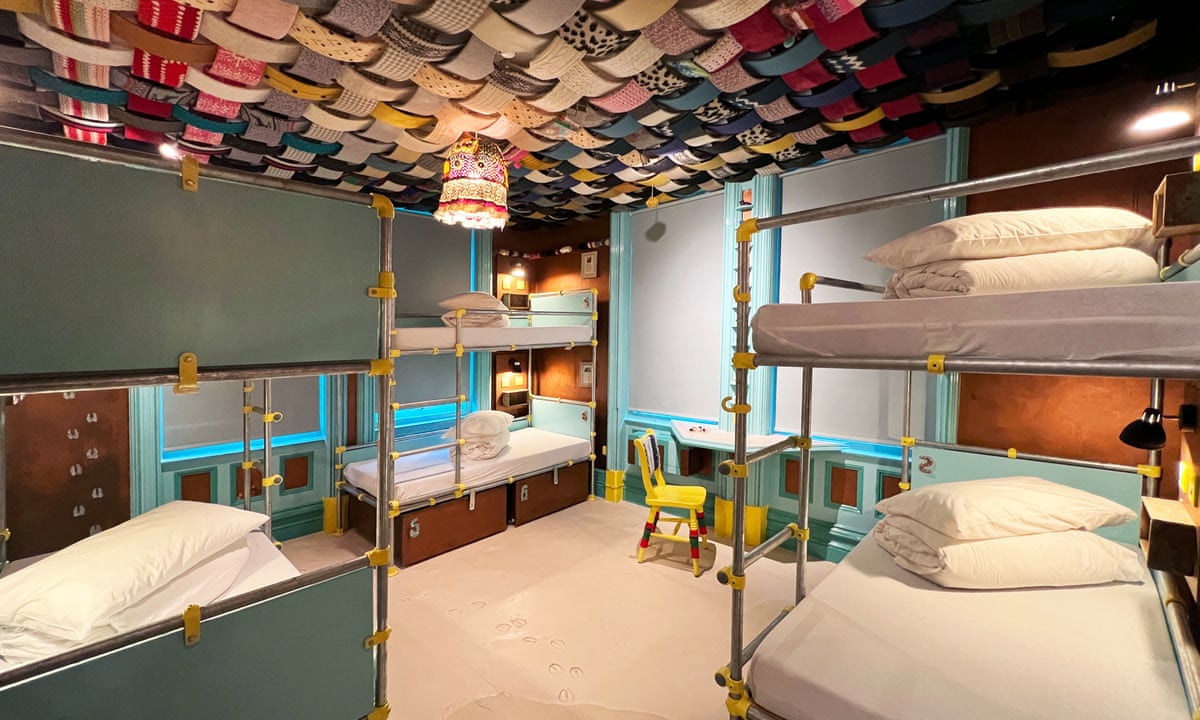The photograph captures the vibrant interior of a children's room, possibly part of a modern school or camp, filled with at least three metal-framed bunk beds situated to the left, right, and back corner of the room. Each bunk bed is a double-decker, equipped with white sheets, pillows, and folded blankets. The beds have distinctive features with one displaying green accents and another red, and numbered for easy identification. The room displays practicality with storage space beneath each bed and individual lights illuminating them. The orange child-sized chair and small desk with a chair add a touch of convenience and coziness.

The ceiling is particularly striking, crafted with a wicker-like weave made from thick strips of multicolored fabric, creating a lively and dynamic pattern. Hanging from this ceiling is an ornate and colorful lamp with a fringed shade, typically suited for tabletop use but creatively suspended overhead. The room's floor is pristine white, adding to the overall brightness, further enhanced by the window shades with bright blue framing. Additional decorative elements include pictures on the walls, contributing to the room's overall cheerful and inviting atmosphere.